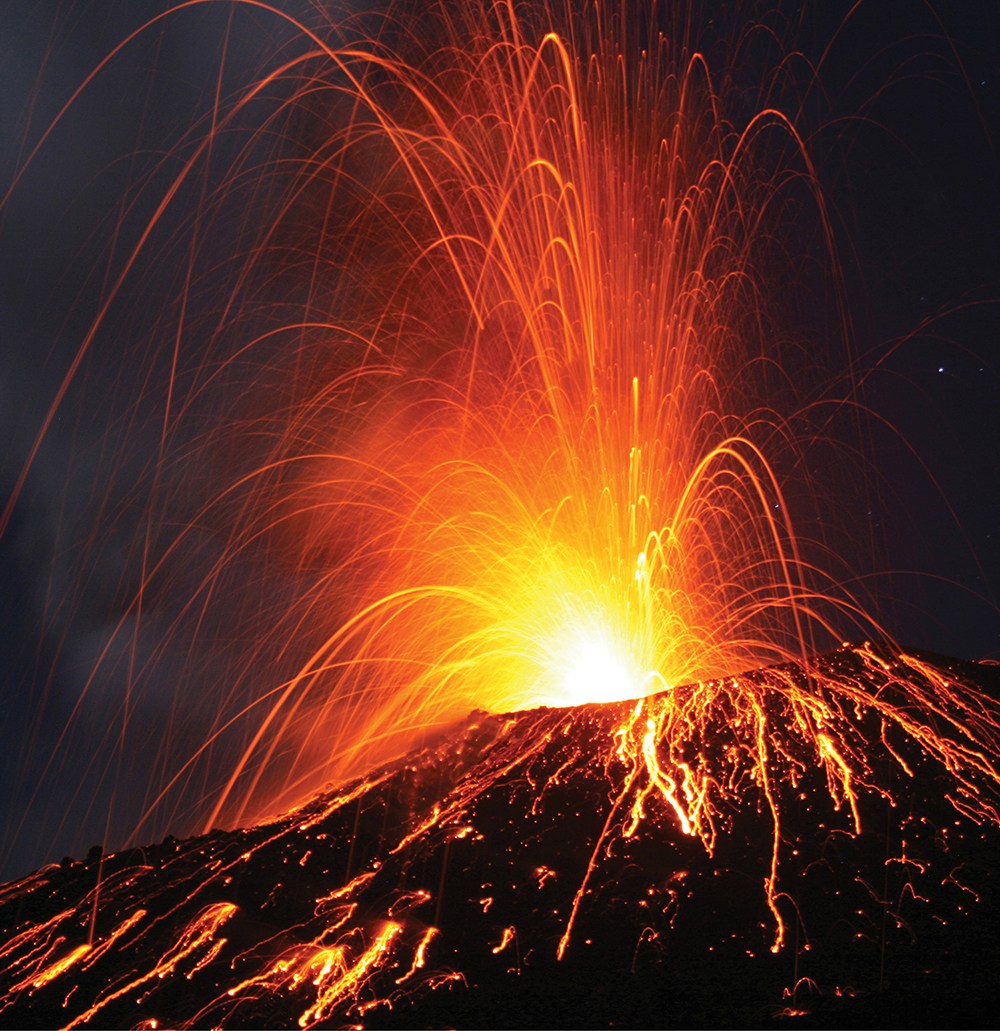This captivating night-time photograph captures the dramatic eruption of a massive volcano in meticulous detail, utilizing a long exposure technique. The volcano’s eruption is mesmerizing with a central core of brilliant white-hot lava that transitions into vivid yellows, deep oranges, and striking reds. The eruption produces thin, hair-like streaks of incandescent debris spewing upward, creating a beautiful gradient of colors that contrasts starkly against the inky black night sky, dotted with a few stars on the right side. Streams of lava flow down the sides of the volcano like glowing veins, adding depth to the mammoth, shadowy silhouette of the mountain. Amid the dark background, this eruption stands out with vibrant strokes of light that trace the path of volcanic fragments, weaving a breathtaking tapestry of natural force and beauty.